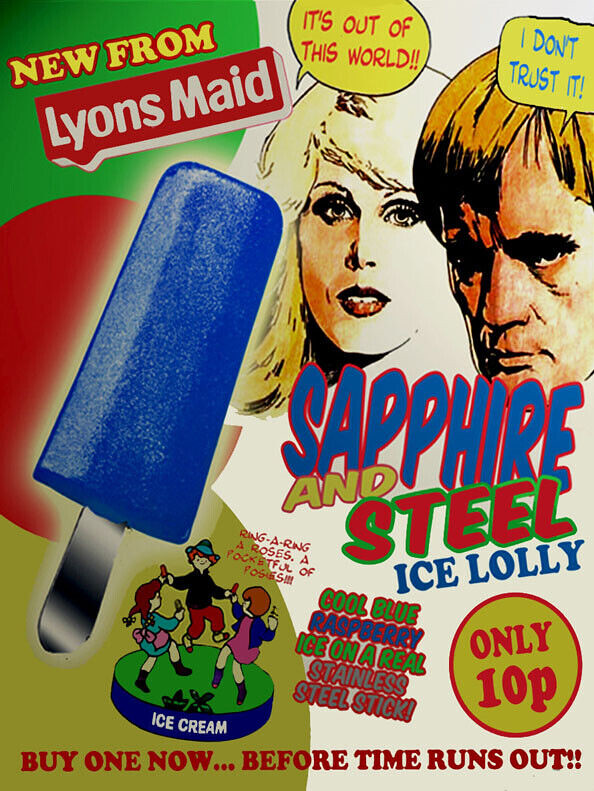This vibrant ad for a Popsicle, styled like a cartoon cover, features a striking blue ice lolly with a unique stainless steel stick prominently displayed in the center left. In the upper left corner, text in yellow reads "New from Lions Made" above a red banner, accompanied by green and red circles behind it. The upper right showcases sketched faces of a blonde woman and a brown-haired man, each with speech bubbles: the woman’s declares, "It's out of this world," in red print on a yellow banner, while the man’s states, "I don't trust it." Below these faces, the product name "Sapphire and Steel Ice Lolly" is prominently written. In the lower left center corner, there's an animated illustration of three children dancing with popsicles, surrounded by text that reads, "Ring a Ring of Roses, Pocket full of Posies," positioned near a logo resembling a green pedestal. To the right of this scene, the ad highlights, "Cool Blue Raspberry Ice on a Real Stainless Steel Stick," and a brown circle indicating the price, "Only 10p." Finally, across the bottom of the ad, a sense of urgency is conveyed with the phrase, "Buy one now before time runs out."